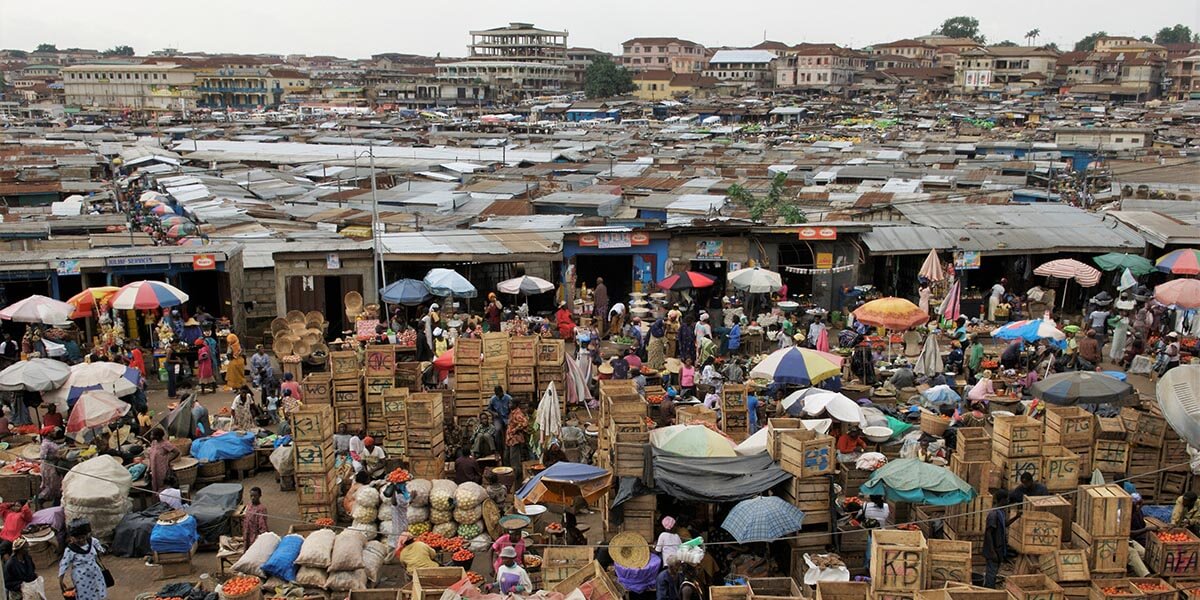The photograph captures a bustling marketplace in what appears to be an African country, seen from a high-angle, semi-aerial view. The foreground teems with activity, dominated by numerous market stalls and colorful picnic-like sun umbrellas providing shade. Around these stalls, people navigate through aisles filled with tall stacks of wooden crates and bags of grain and vegetables. The vendors and patrons, dressed in traditional African attire, add to the vibrant atmosphere. In the mid-ground, a row of storefronts is visible, with more people engaged in commerce. Beyond this, the background transitions into a densely packed array of flat-topped, side-by-side buildings that stretch out for miles. The scene lacks modern infrastructure such as skyscrapers or highways, further reinforcing its setting in a developing region. The skyline is almost white, with just a few trees rising above the taller buildings in the distance, indicating a clear, bright day.